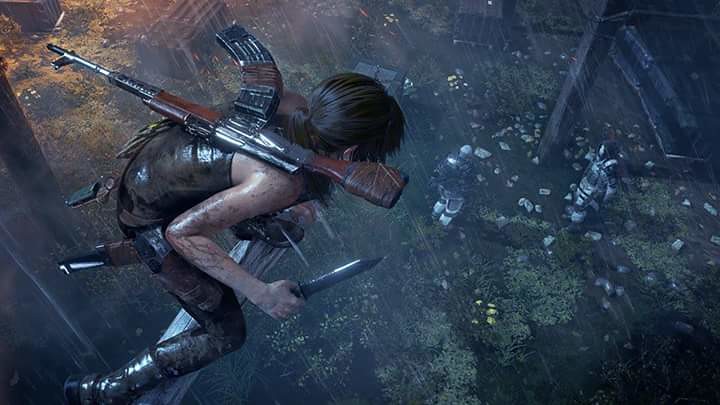A computer-generated screenshot from a video game displays a side-view angle of a small woman crouching on a rooftop, looking down intently. She leans forward, revealing a machine gun strapped to her back and a knife clutched in her hand. Her white skin is marred with dirt or veins, and her brown hair is visibly damp from the rain. To her left, a field stretches out, dotted with wild grass and a lone crate. Beneath the support beam of another structure, two figures in suits or armor converse; one wears a hood while the other does not. The woman observes them closely, her position and weapons suggesting she is preparing for a stealthy action.